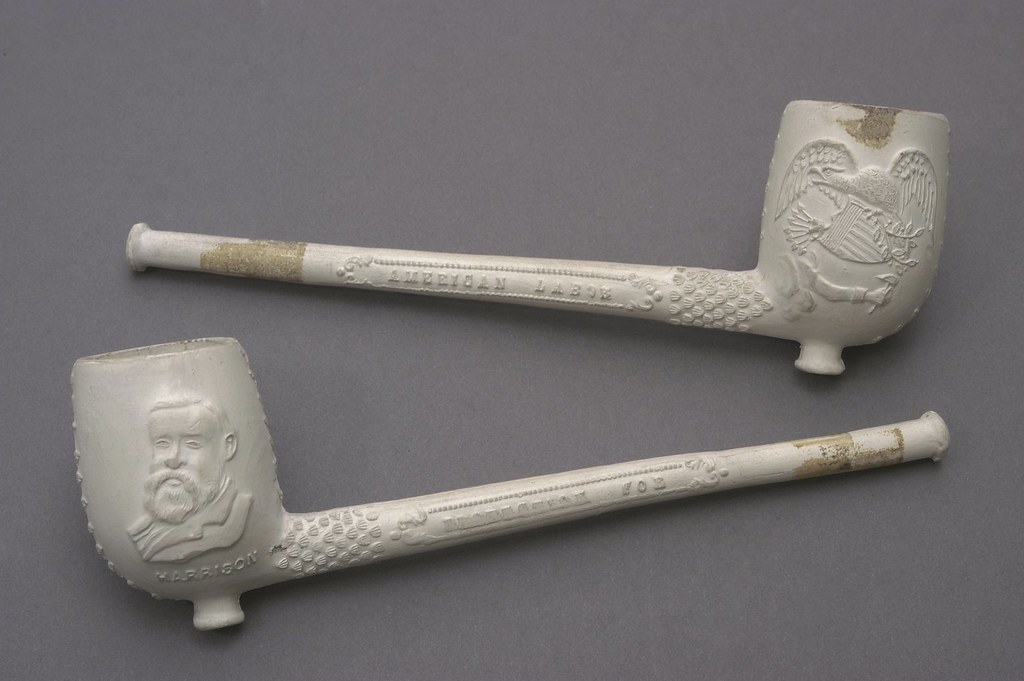This is a photograph featuring two old-fashioned smoking pipes, each with intricate engravings and positioned one above the other on a grayish-blue surface. The pipes are likely made of clay and have a white color. The top pipe, with the bowl on the right and the stem on the left, displays detailed carvings including a central shield motif above which spreads the wings of a bird, presumable an American bald eagle. Beneath the shield, a person is depicted holding an indistinguishable object. Along the stem, the text "American Labour" is partially visible. The bottom pipe, oriented in the opposite direction with its bowl on the lower left, bears the engraved image of a man with a mustache and beard wearing a collared jacket. Below this portrait, the name "Harrison" is inscribed, likely referring to President Harrison. Both pipes exhibit additional fine engravings resembling scales or lines, contributing to their historical character and craftsmanship.